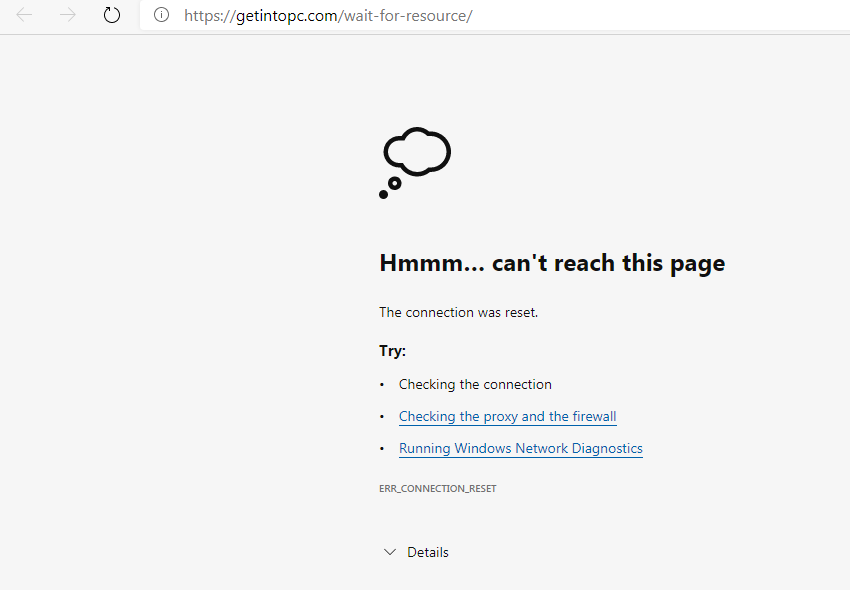The image is a screenshot of a web browser error message. At the top of the browser, the URL https://getintopc.com/wait-for-resource/ is displayed. Below the URL, there is a message with an illustration of clouds at the top, stating "Hmm… can't reach this page." 

The error message further explains that "The connection was reset," and suggests the following troubleshooting steps:

- Checking the connection
- Checking the proxy and the firewall (This option is clickable and underlined in blue)
- Running Windows Network Diagnostics (This option is also clickable and underlined in blue)

At the bottom of the message, in smaller capital letters, the error code "ERR_CONNECTION_RESET" is displayed. To the left, there is a downward-facing arrow, and next to it, in black text, the word "Details" is shown.